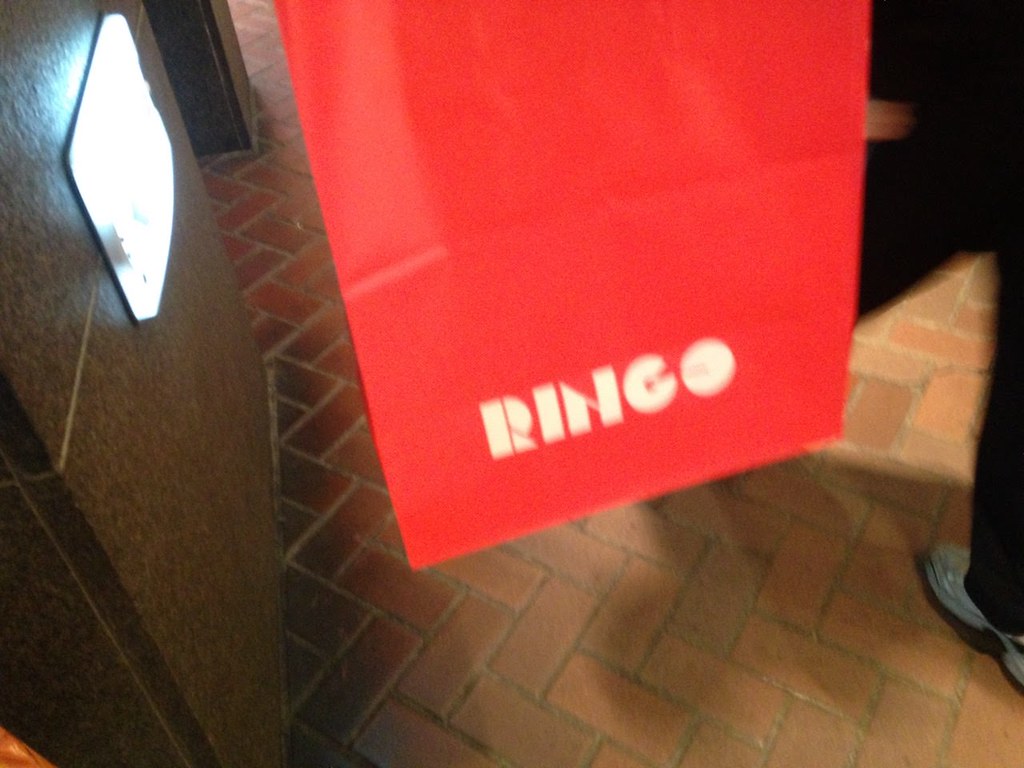The photograph, slightly out of focus, captures an indoor setting that appears to be a restaurant or similar establishment. Central to the image is a small red banner hanging downward, emblazoned with the word "RINGO" in a stylized white capital font. The banner extends upward beyond the frame. The floor beneath features a red brick herringbone pattern. On the left side of the image, there is a brown tiled wall with a light mounted close to the floor, presumably illuminating a nearby gap that looks like a doorway. Towards the right, a person is partially visible, wearing black pants and gray tennis shoes, seemingly in mid-walk. An orange object is faintly noticeable in the far left corner of the image.